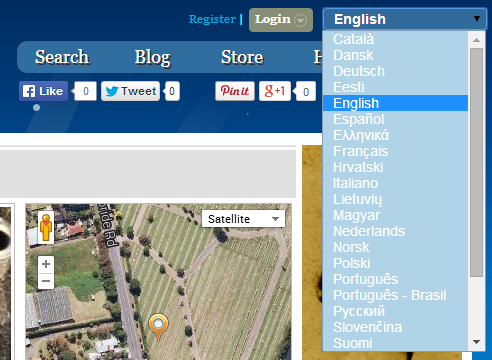At the top of the website, the background features a gradient from blue to a lighter blue shade, with a prominent "Register" button. Adjacent to it, there's a gray rectangle with the word "Login" in white text. Below, an outlined gray circle and a downward-pointing gray triangle are visible, indicating a dropdown menu. 

A rectangular scroll bar, colored in bluish hues, runs along the right side with a black rectangle embedded within it. At the very top, "English" is displayed in white text, accompanied by a dropdown menu offering additional languages, such as "Español" (Spanish) and "Français" (French).

Beneath this is another gray rectangle in a different blue shade, prominently featuring the white text "Search Blog Store." Due to the scroll position, additional content is partially obscured.

Below this, several interactive elements include:
- A Facebook Like button with a white box and a black '0'.
- A gray box with a "Tweet" label next to a blue bird icon.
- A white box displaying a black '0'.
- A white rectangle with "Pin it" written in red.
- Another white rectangle labeled "G plus one" in red.
- A white box containing a black '0'.

The background transitions to white and then to gray towards the bottom. The right side of the screen is blocked out, while the left side features a visible map.